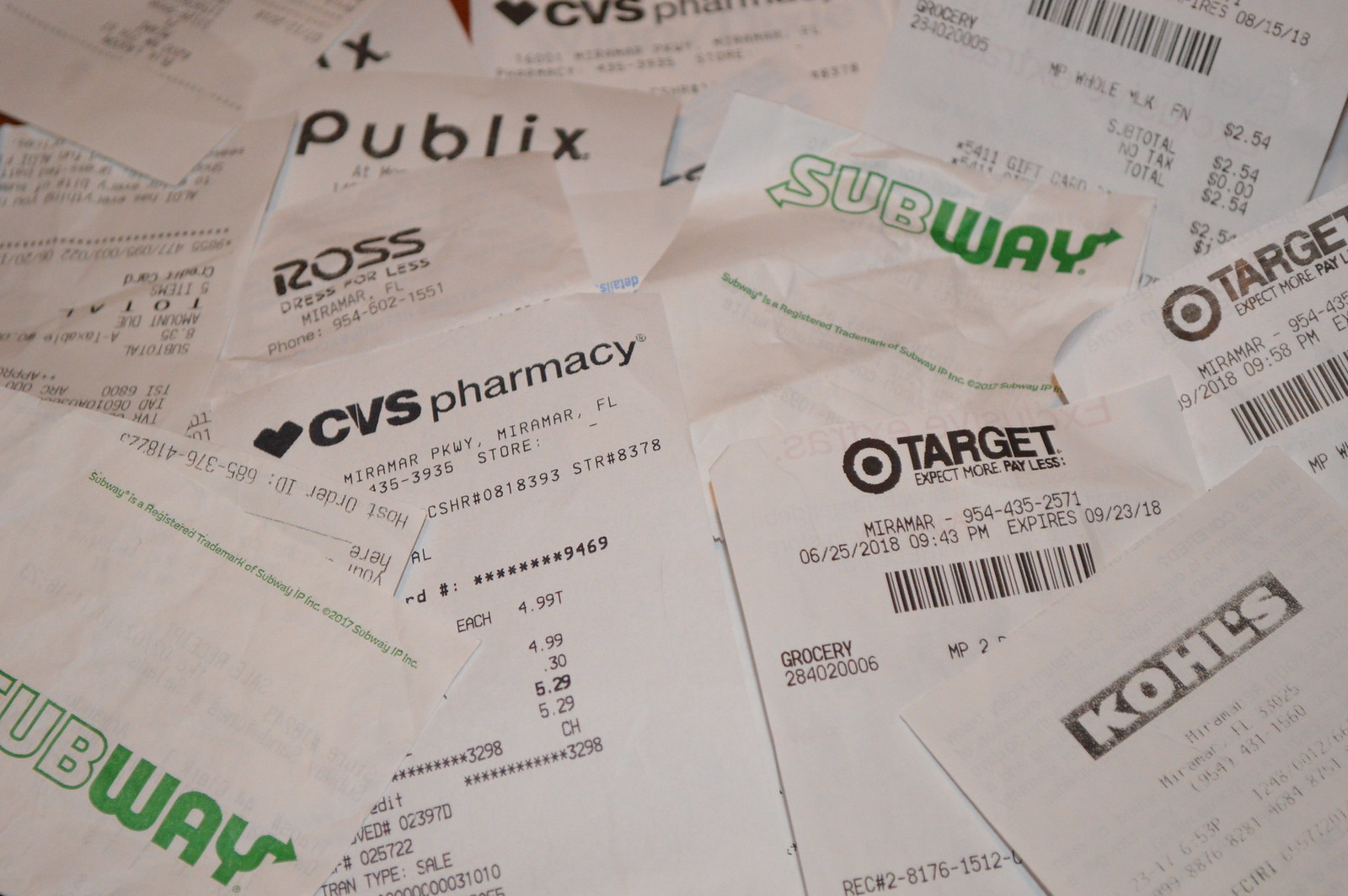The image features a densely layered pile of white paper receipts, predominantly displaying black text. The receipts overlap one another, creating a chaotic but detailed array that obscures the background except for small glimpses of red in some areas. Key elements include two prominently placed Subway napkins with the Subway logo in green text, positioned centrally and at the bottom left-hand corner. Among the various receipts, notable ones are from stores in Miramar, Florida, including Kohl's, Target, CVS Pharmacy, Ross Dress for Less, and Publix. A CVS receipt in the foreground shows a total of $5.29, while another receipt towards the back lists grocery items including milk priced at $2.54. Most of the receipts are slightly out of focus but collectively suggest a recent shopping spree in the Miramar area.